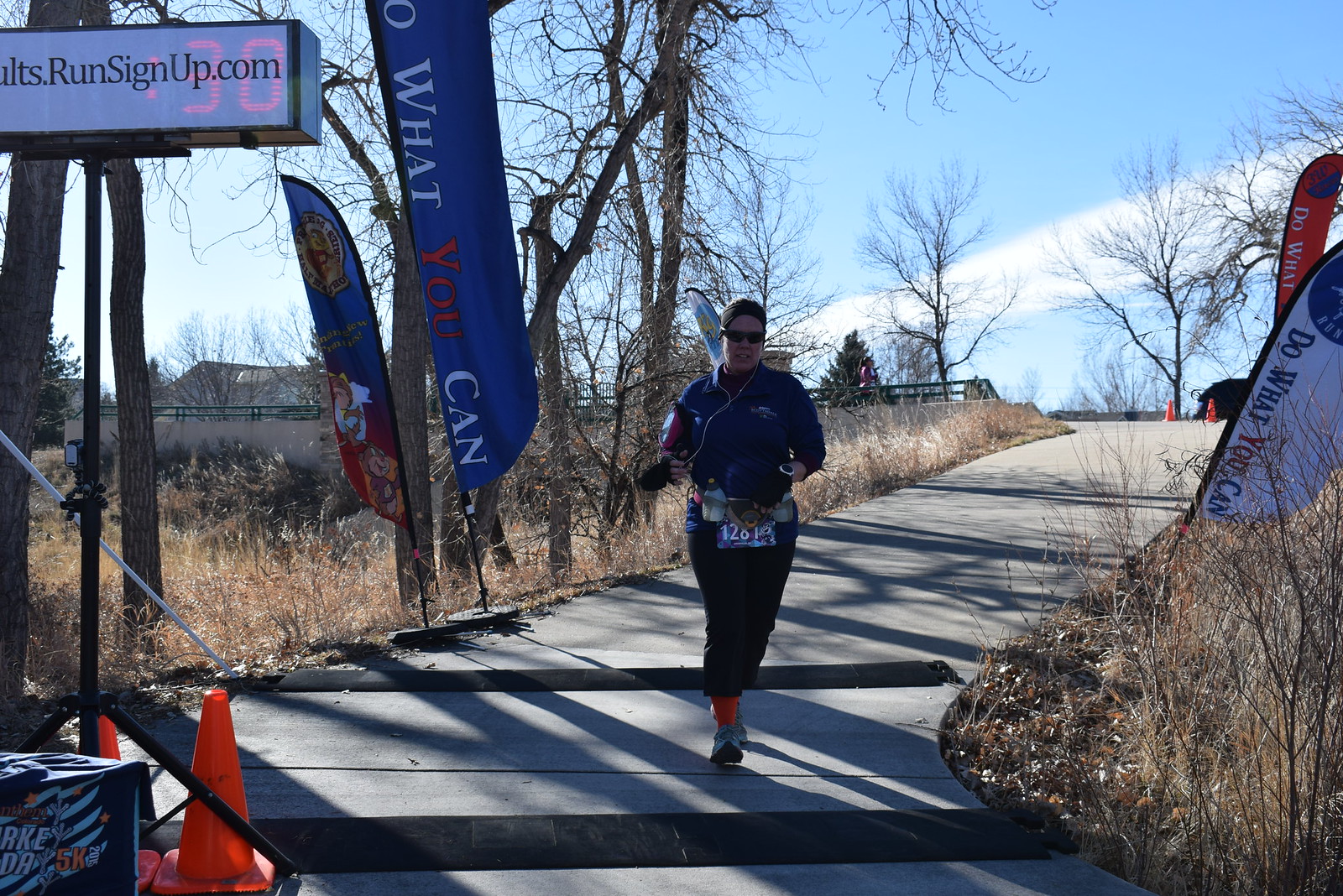The image captures a dynamic moment of a race, featuring a female runner in the center, poised to place her right foot down on a sloping concrete path. She is looking directly at the camera with a smile, wearing sunglasses and a black headband. White earphones with a visible cable running to an armband device accompany her blue, body-hugging top, which bears a white label. Her outfit includes black trousers, orange socks, and trainers.

Around her waist, she sports a utility belt holding a water bottle and accessories, along with a race bib partially visible with the number "1281". The runner is clearly in motion, captured running downhill on a path that is framed by barren trees and brown grass, indicative of a winter setting.

Flanking the path are a series of banners with motivational text, including vertical ones reading "Do what you can," and an orange cone positioned in the bottom left of the frame. Further in the scene, a sign displaying "runsignup.com" is visible, set within a light box showing "30" in red. The sky above is clear and blue, enhancing the sense of accomplishment and joy as the runner approaches what appears to be the finish line, indicated by her imminent step across a black pad.